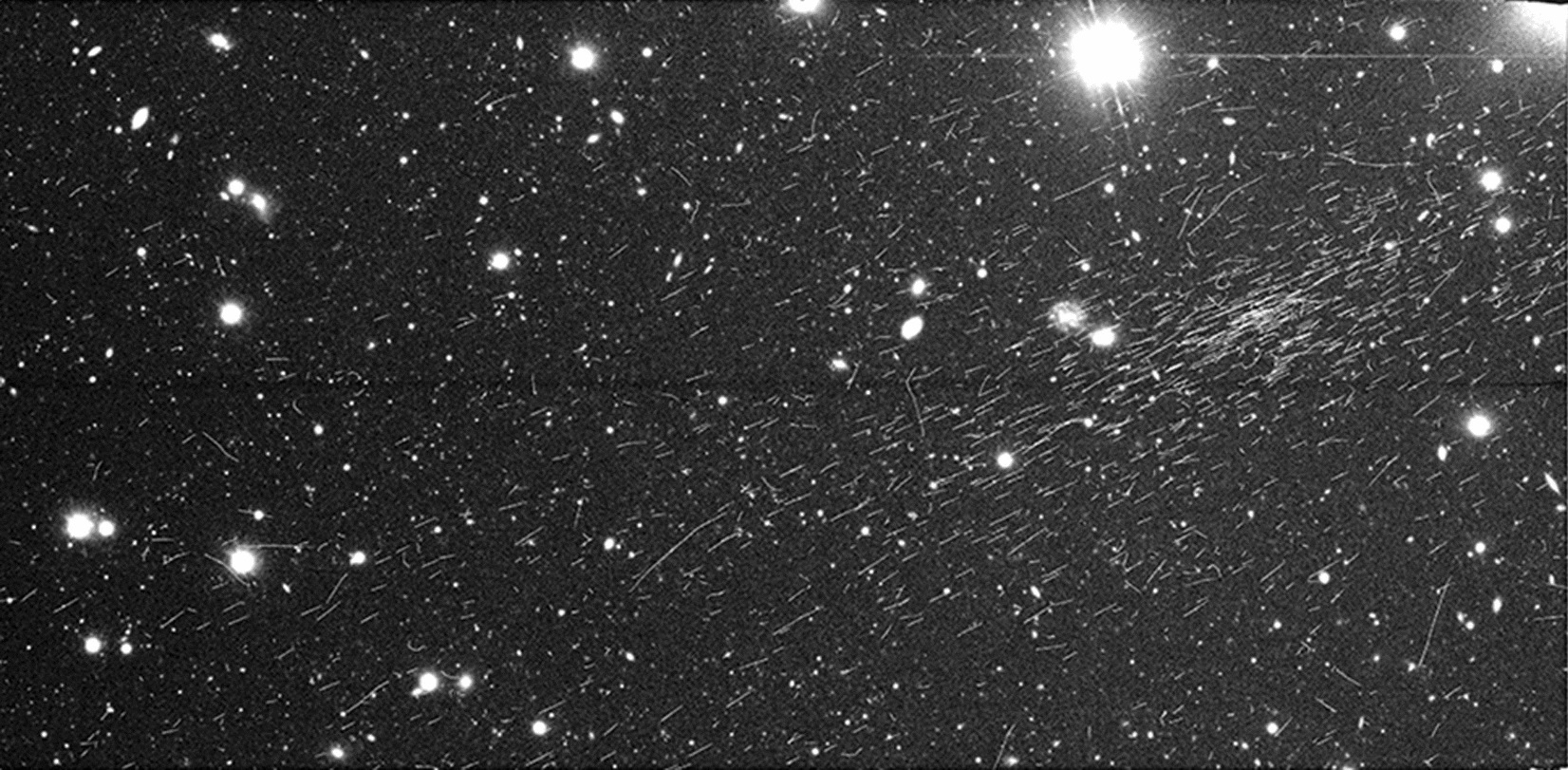This image presents an enigmatic, abstract artwork featuring a black background with splashes and lines of white scattered throughout. It evokes curiosity and multiple interpretations, resembling either a night sky with stars, an abstract photograph, or perhaps an image captured under a microscope. The composition includes larger glowing orbs, some about the size of a dime, and smaller specks akin to tiny stars or sparks. The white lines vary in length and appear randomly arranged, at times resembling hair trimmings or patterns seen through a telescope. Overall, the artwork is divided into two halves, each mirroring the other, enhancing the mysterious and creative essence of the piece.